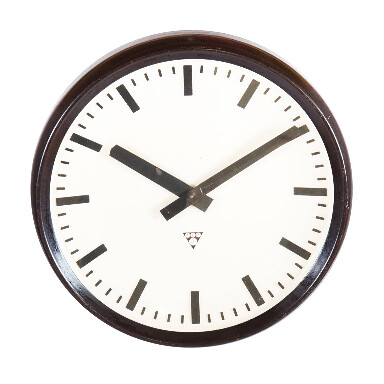The photograph captures a round, analog wall clock set against a completely white, backgroundless backdrop, much like a stock photo. The clock's frame is composed of a polished, dark wood that appears black or deep brown, thicker toward the top and tapering to a thinner section at the bottom, giving it a unique asymmetrical border. The inner frame, subtly separated yet similarly colored, adds an extra layer of detail to its design. The face of the clock, with an off-white hue, features thick, black rectangular dashes to indicate the hours, while smaller, thinner dashes mark the minutes. The hands of the clock are also black and rectangular, with the longer minute hand pointing at the 10 and the shorter hour hand at the 2, setting the time to 10:10. Below the clock hands, a small triangular segment with a few white dots is visible, adding a touch of distinctiveness to the clock's minimalist design.